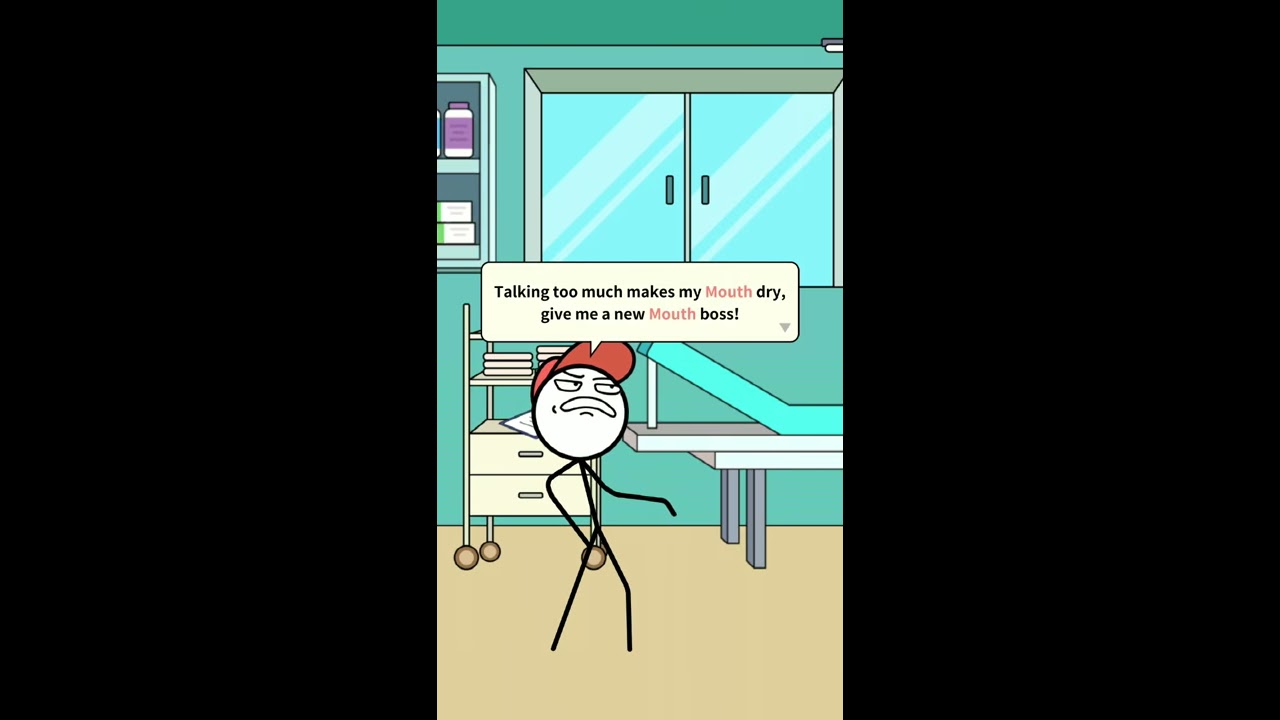This digital cartoon image depicts a stick figure wearing a red baseball cap in a doctor's office. The scene is set against an aqua-colored wall, with the stick figure positioned slightly off-center towards the bottom left. To his right, a white and gray patient table with aqua accents stands beneath a light blue window, which shows reflections on its glass. Behind the figure is a tan wheeled storage unit, and above it, a cabinet with a purple pill bottle inside. The tan floor adds a neutral base to the scene. Text above the figure says, "Talking too much makes my mouth dry, give me a new mouth boss," with the word "mouth" highlighted in red. Black bars frame the left and right sides of the image, enhancing its comic-style presentation and making the humorous caption more impactful.